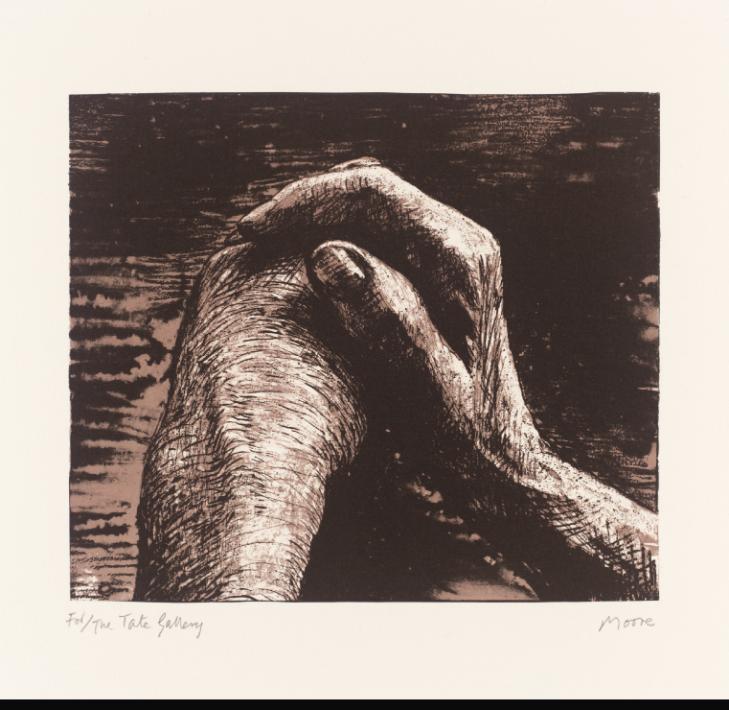This is an intricate drawing by Henry Moore titled "Hands 1," created in 1973. The artwork, encapsulated in a square format and inset into a cream-colored mat with the artist's signature on the bottom right corner, depicts a detailed and textured sketch primarily in off-white and brownish black hues. Two hands dominate the composition; the right hand, appearing elderly with visible wrinkles and characterized by its prominent thumb and index finger, rests over the partially obscured left hand. The left hand's thumb and some fingers are partially visible beneath the right hand. Both hands are shown from the wrists to the fingertips. The background features an abstract, wavy pattern resembling a piece of wood or a wet tabletop, enhancing the modernist style of the piece. The overall scene is set against a muted background of dark brown and black tones, adding depth and contrast to the meticulous renderings of the hands.